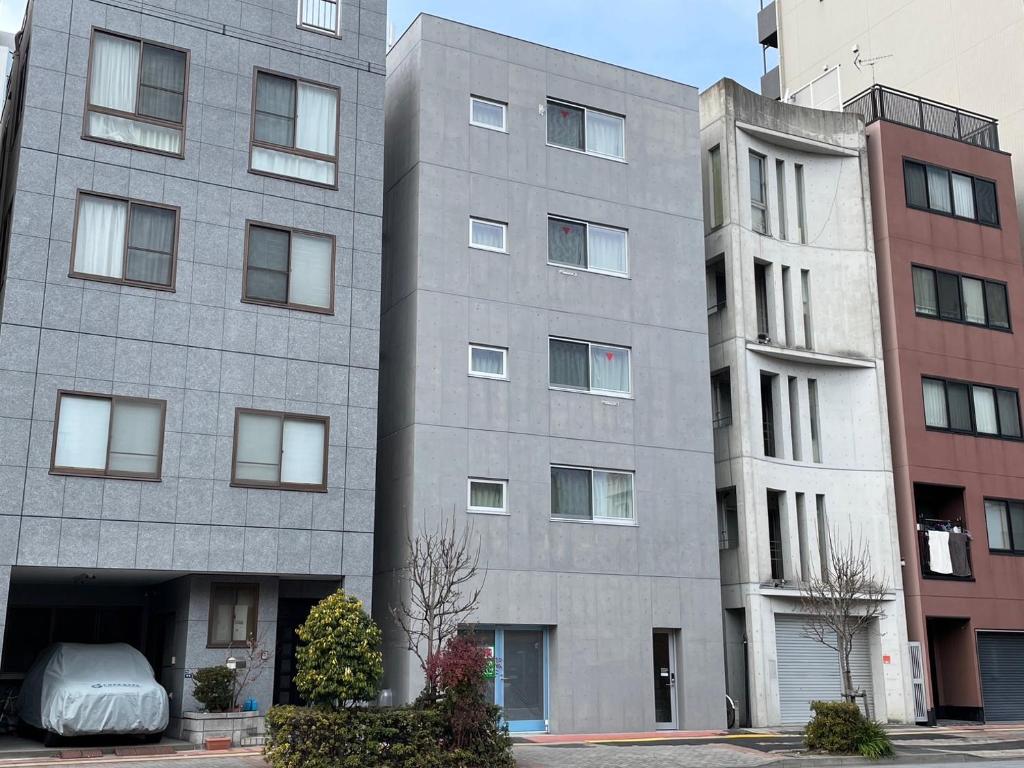This photograph captures a row of four narrow, tall apartment buildings, each featuring distinctive architectural details. The far left building is clad in gray slate tiles with three visible stories, each hosting two windows. At its base, there is an entrance with a covered car parked inside and nearby, a small square hedge with a tree and a dormant tree with bare branches. The next building to the right is a lighter, warmer-toned gray and has four stories with a mix of smaller left-side windows and larger right-side windows. It features a blue glass double door and a smaller single-pane glass door at ground level. Adjacent is a very slender white building, half the width of its neighbors, adorned with four rows of thin windows and a shuttered door at the bottom. Finally, the rightmost building stands out with its burgundy façade and wide black-framed windows spanning nearly the entire width of each floor. It also has a black shuttered door on the ground floor and entry corridors on both sides. The buildings are well-maintained, and the presence of trees and shrubs in front adds a touch of greenery. The image, taken during daylight under a clear sky, also shows taller buildings in the background, indicating a dense urban environment.